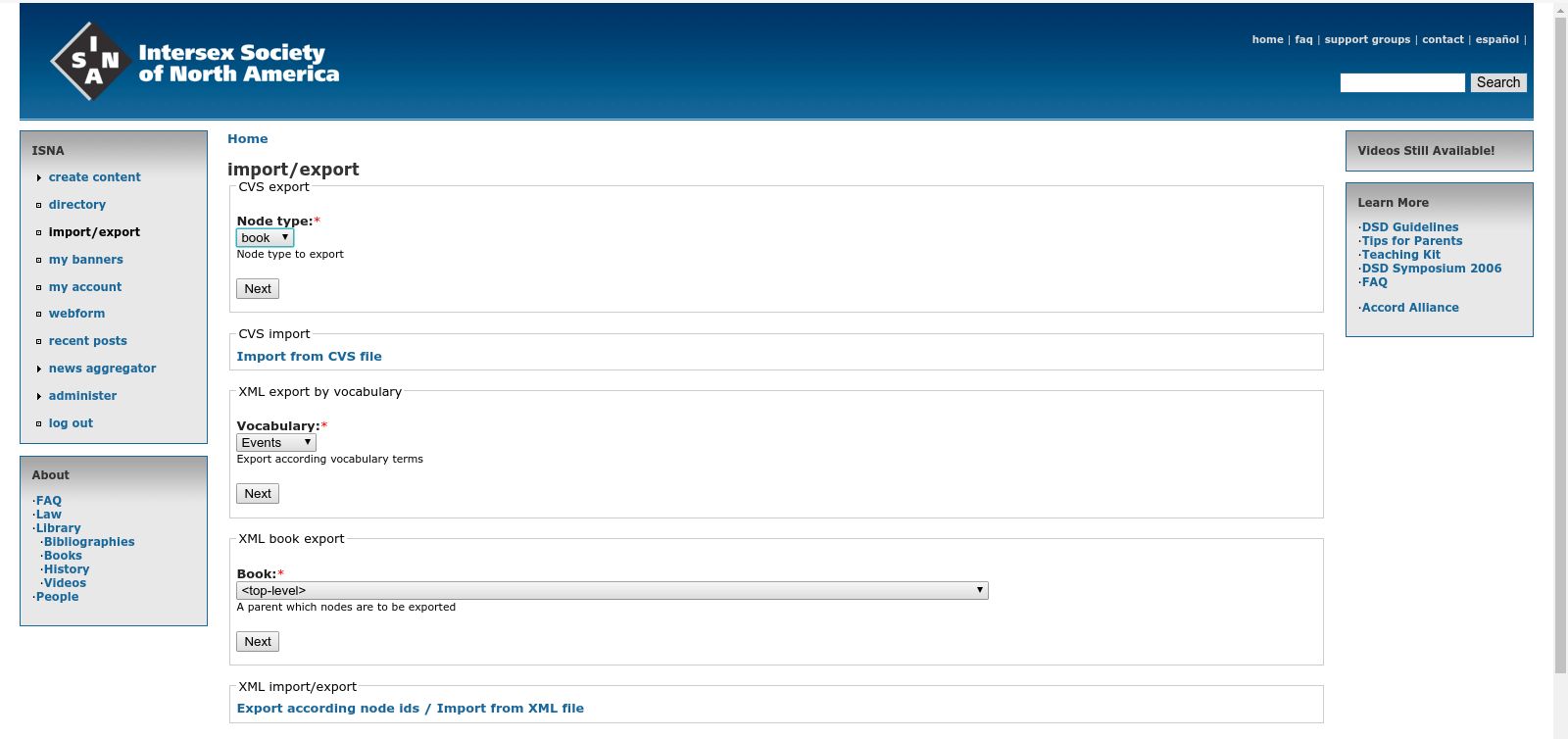Detailed Caption: A cropped screenshot of the import-export page of the Intersect Society of North America (ISNA) website. The top header is dark blue, featuring the ISNA logo on the left side, which is a diamond shape with "ISNA" inscribed in white letters. To the right of the logo, "Intersect Society of North America" is prominently displayed in large white font. Further to the right, a series of site categories—Home, FAQ, Support Groups, Contact, and Español—are listed in small white letters. At the far right end of the header, there is a small search box with a gray search button adjacent to it.

Below the header, to the left side of the page, there are two gray boxes with blue outlines. The top box has "ISNA" in bold black letters, followed by a vertical list of subcategories: Create Content, Directory, Import-Export, My Banners, My Account, Web Form, Recent Post, News Aggregator, Administer, and Logout. The "Import-Export" subcategory is selected, indicated by a highlighted state in the list.

The main content area, which is open to the "Import-Export" section, has a white background. At the top of this section, "Home" is written in bold blue letters, followed by "Import-Export" in bold black letters. Below that, a series of long rectangular boxes contain various import-export functions. 

The first box is labeled "CSV Export" in small black letters. Directly below this, the words "Node Type" in bold black letters are followed by a red asterisk, indicating a required field. A drop-down box below shows the current selection as "Book." Under this, it says "Node Type to Export" in small black letters. A gray "Next" button is located at the bottom left of this section.

Next is the "CSV Import" box. Following this is the "XML Export by Vocabulary" box, which includes a drop-down menu labeled "Vocabulary," currently set to "Events." 

Further down, the "XML Book Export" box includes a drop-down menu set to "Top-Level." A "Next" button appears at the bottom left of this section. 

The final box is labeled "XML Import-Export." Within this box, blue text indicates two options: "Export according to node IDs" and "Import from XML file."